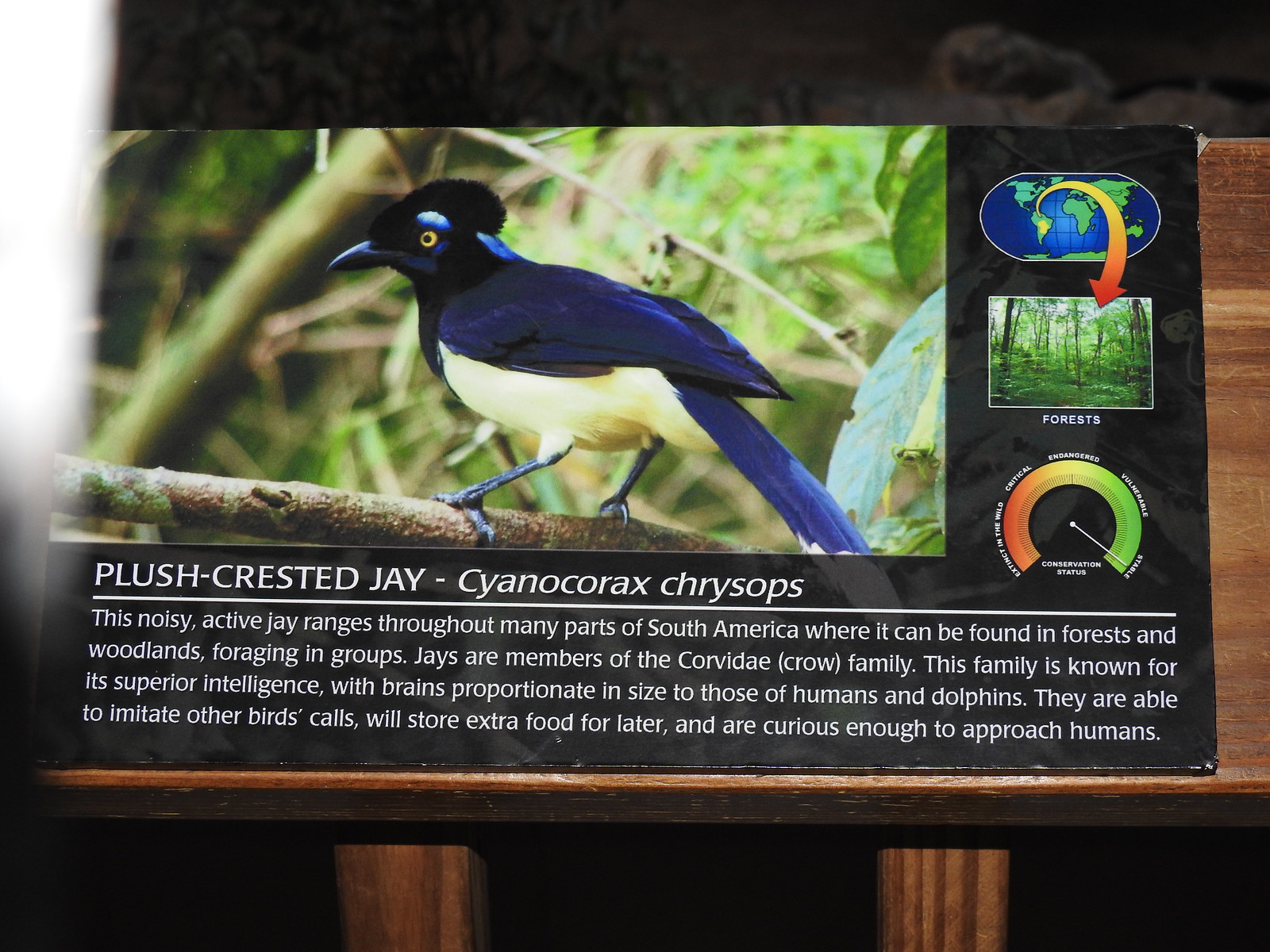The image depicts a detailed wooden information sign, supported by wooden posts, likely situated in a zoo or wildlife preserve. The sign features a prominent illustration of a plush-crested jay (Cyanocorax chrysops) occupying about three-quarters of the space, starting from the top left corner and extending across the sign. The bird, characterized by its dark blue wings, blue tail, white underbody, black claws, black head plume, yellow eye, and distinctive beak, is shown perched on a branch.

Beneath the illustration, a detailed description outlines that the plush-crested jay is a noisy and active bird found throughout many parts of South America, particularly in forests and woodlands. It is part of the corvidae family, known for superior intelligence with brain sizes proportionate to those of humans and dolphins. These birds are noted for their ability to imitate other birds' calls, their behavior of storing extra food, and their curiosity, which often leads them to approach humans.

On the upper right side of the sign, an oval global map projection indicates the bird's native range with an arrow pointing to the respective forests. Another circle below the map provides additional information about the bird and its habitat.